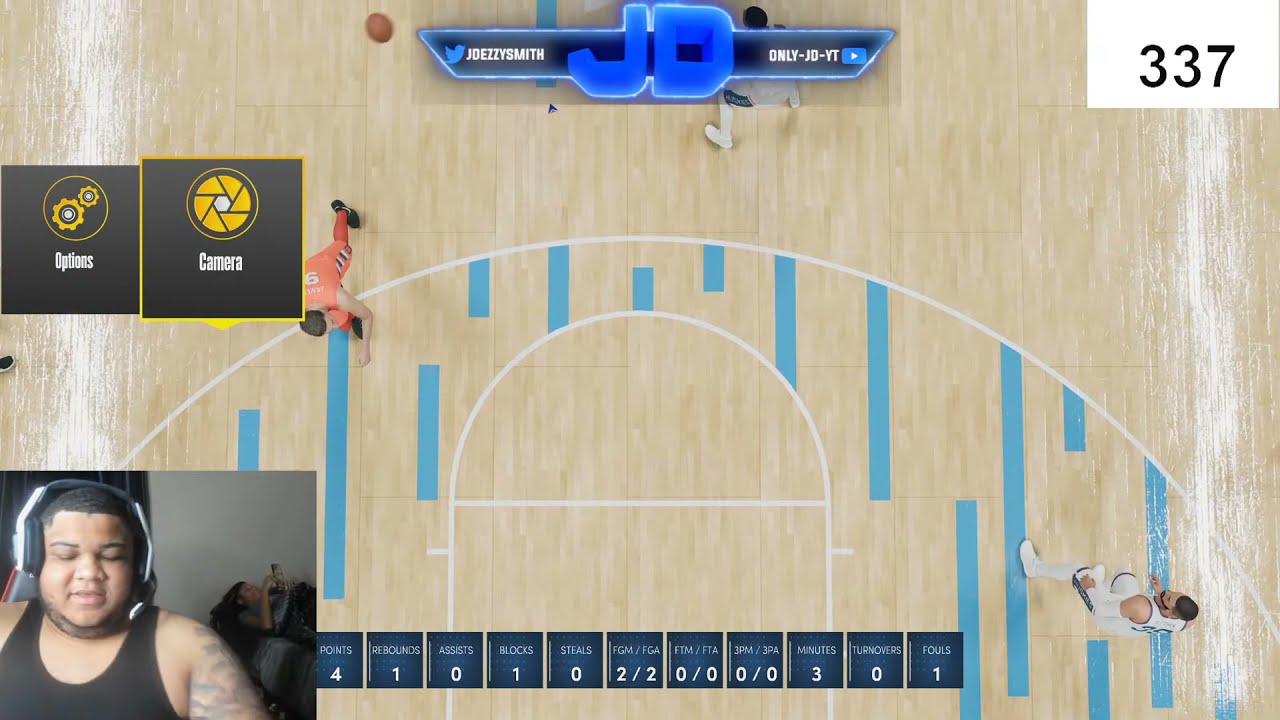The image captures an immersive moment within a basketball video game. Dominating the scene is an overhead view of a realistic basketball court characterized by its light brown wooden floor with blue vertical stripes inside the three-point arc and the free-throw line. On the court are players in distinct uniforms: two players sporting white and blue, positioned at the bottom right and the top middle, and another player in an orange jersey with black and white stripes on the left. The basketball is visible, though not in active play.

Overlaying the game, textual elements include a banner at the top displaying "JD" in large blue letters. On the left side of the banner, a Twitter symbol beside the name "JD Ezzie Smith" is visible, while on the right, the name "only-JD-YT" is accompanied by a YouTube icon. Additional in-game graphics include stats at the bottom of the screen and a small white rectangle in the upper right corner displaying "337."

In the bottom left corner, a live streamer is visible, inset within the main image. The streamer, a young black man with tattoos on his left arm, is wearing a black tank top and a headset. His mouth is slightly open, suggesting that he is speaking or possibly reacting to the game. Above his image are two black boxes: one labeled "options" with a yellow gear icon and the other labeled "camera" with a yellow camera lens icon. Slightly behind him, a woman lies on a couch, appearing disengaged as she focuses on her phone.